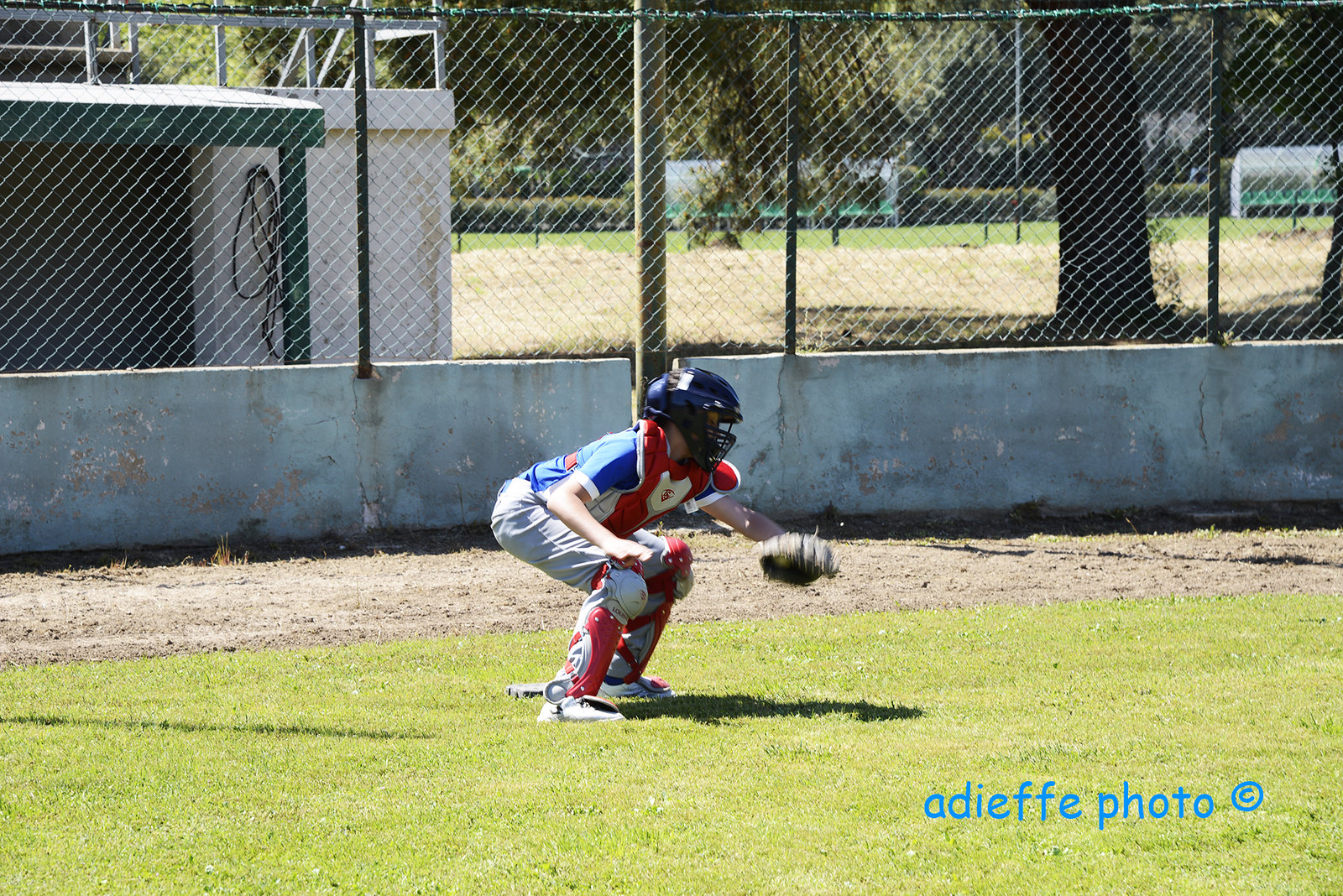This wide rectangular image captures a young baseball catcher, poised in the center of a green, shortly trimmed grass field, which transitions into a band of brown dirt as it extends slightly diagonally upwards. The child, appearing small and suggesting a youth game, is donned in detailed red and gray catching gear, including a blue helmet, a red vest, red shins, gray pants, and white knee-length pants. His white sneakers are firmly planted in the grass as he crouches low, almost horizontal, in a classic catcher’s stance. His gloved hand is raised and slightly blurred, indicating possible motion as he anticipates a pitch. In the background, a chipped light blue barrier and gated fence mark the edge of the field, leading into what appears to be a dugout. Beyond, scattered sports fields and a white building resembling bleachers complete the scene. In the bottom right-hand corner, blue lettering reads "a DFA photo" accompanied by a copyright symbol, hinting at the image's professional nature and artistic style.